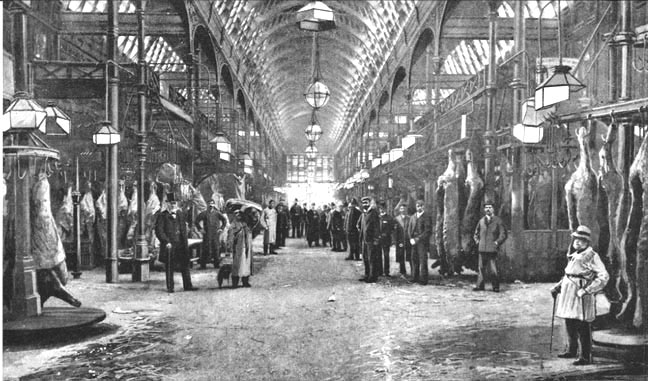This black-and-white, borderless photograph depicts the interior of a large industrial-era warehouse or stockyard, possibly from the 1920s. The building has high, arched ceilings that reach up to three stories, adorned with various hanging lights and antique lampshades. In the center of the image, numerous people are gathered, many of whom are men dressed in suits, bow ties, and top hats, possibly indicating their roles as owners or supervisors. Among them are women wearing dresses and bonnets, with one woman noticeable at the lower right corner holding a cane. Scattered throughout the space are several columns sectioning off different areas of the warehouse.

The ground appears to be composed of dirt and rocks, adding to the industrial atmosphere. Hanging from the ceiling and walls are numerous hooks and railings bearing the carcasses of cows and other meats, indicative of a meat market or butchery. To the far right and left, animal skins and meat cuts dangle, contributing to the scene's authenticity. At the end of this broad hallway, an open garage door allows light to stream in, illuminating the bustling activity below and suggesting an exit point from the facility.